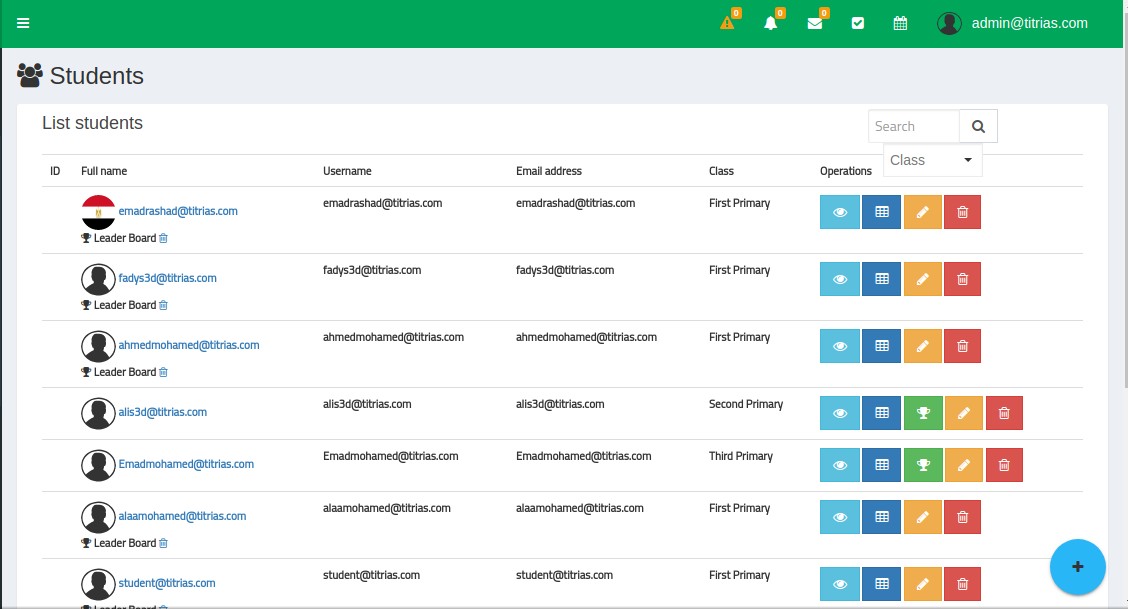Detailed Caption:
The image depicts a teacher-oriented software interface designed for tracking student progress, displayed in landscape mode, likely on a laptop or desktop monitor. At the top, a green navigation bar stretches across the width of the screen. On the far left of this bar is a menu icon represented by three stacked white lines. On the far right side, there's a user silhouette icon followed by an email ID in the format of admin@[something].com. Next to the email ID, the company name appears to be TITRIS, although the exact spelling is unclear (possibly T-I-T-R-I-S). To the right of the company name is a row of interactive icons, including an envelope icon with a message count, an alert or alarm icon, and a calendar icon.

Beneath the green bar, the background transitions to a pale blue shade. The section title "Students" is prominently displayed, accompanied by an icon of three people, suggesting group management features. On the left side, there's a white button labeled "List Students." On the top right of this subsection is a search bar with a class drop-down filter underneath it, allowing for refined searches.

The main content area lists students' details in several columns: Names, Usernames, Email Addresses, Classes, and Operations. The Operations column includes various icons for possible actions: an eyeball for viewing details, an unclear second icon, a pencil for editing, and a trash can for deleting entries. Additionally, two of the student entries feature a fifth icon— a green square with a white trophy symbol, likely indicating awards or achievements for those students.